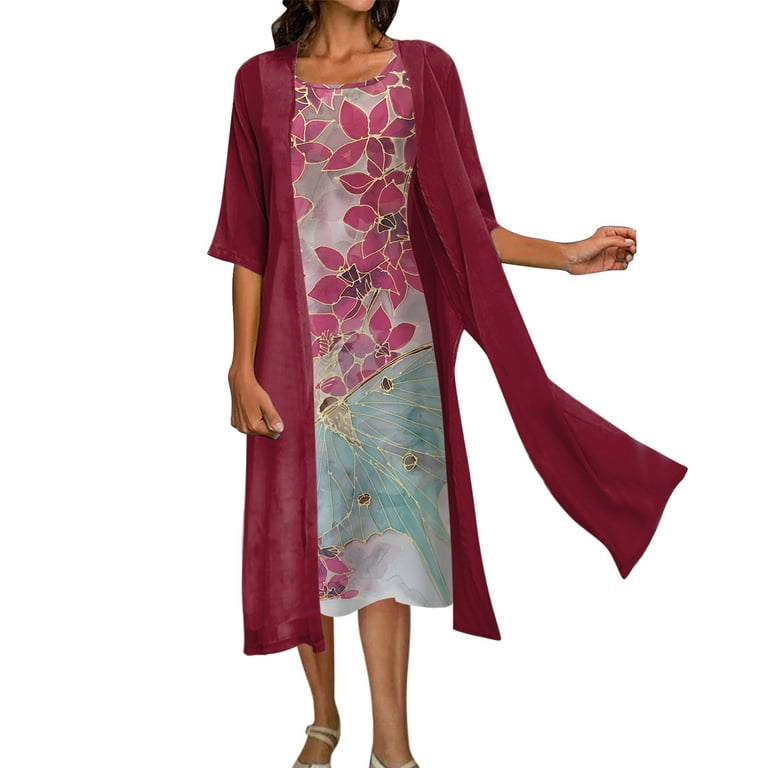The image showcases a woman with slightly darker skin and long brown hair, set against a solid white background. Her face is partially visible, ending just below her chin, and her feet are mostly shown except for her toes, which are cut off. She is dressed in a floral print gown adorned with large dark pink petals outlined in gold on the upper body, transitioning into angled gold lines with some green shading from the waist to the knees. The gown stops just below her knees. She wears white high heels that slightly blend with her skin tone. Over her gown, she dons a silky, dark red robe that drapes elegantly on both sides and billows slightly. Her right arm hangs down by her side with her fingers curled, while her left arm extends outward, poised as if about to grasp something. This fashion image emphasizes the contrast of her vibrant attire against the stark white background.